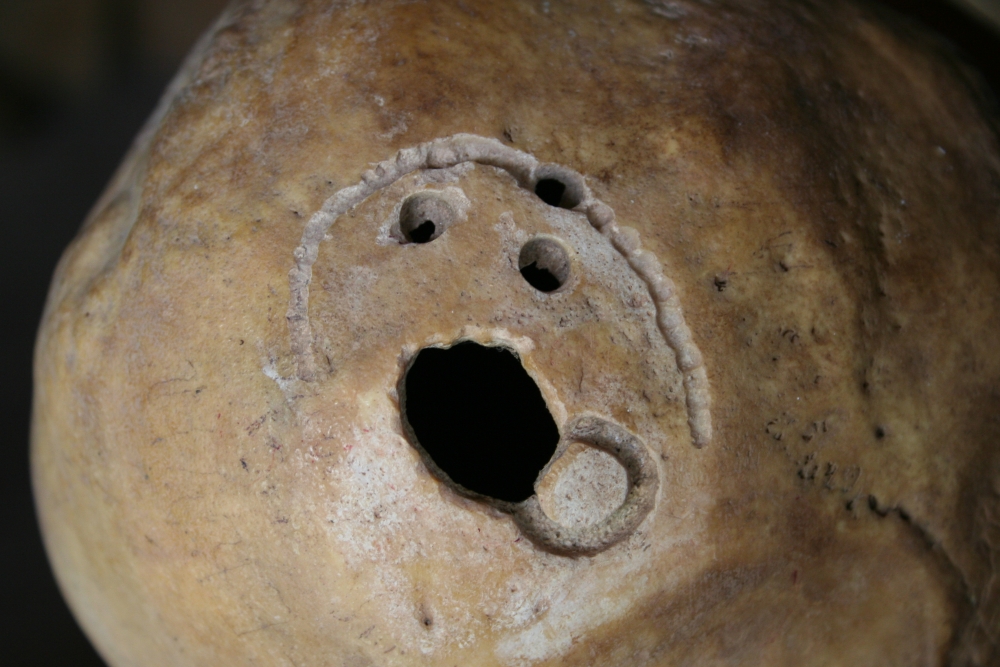Against a very dark background, a close-up photograph features a stone or skull-like object that is prominently brown and beige, with various shades and speckled black sections, suggesting wear and age. The stone has numerous cracks and grooves, adding to its worn appearance. Central to the image are several holes that form a notable pattern: three small holes arranged at the top, resembling a bowling ball's indentations, and a larger, deep hole slightly below the middle, where the black interior is visible. Surrounding these holes is a semicircular groove, giving the impression of a smiley face with two eyes and an open mouth in an "O" shape. The detailed carvings and indentations, along with the stone's texture, accentuate its aged and unique appearance.